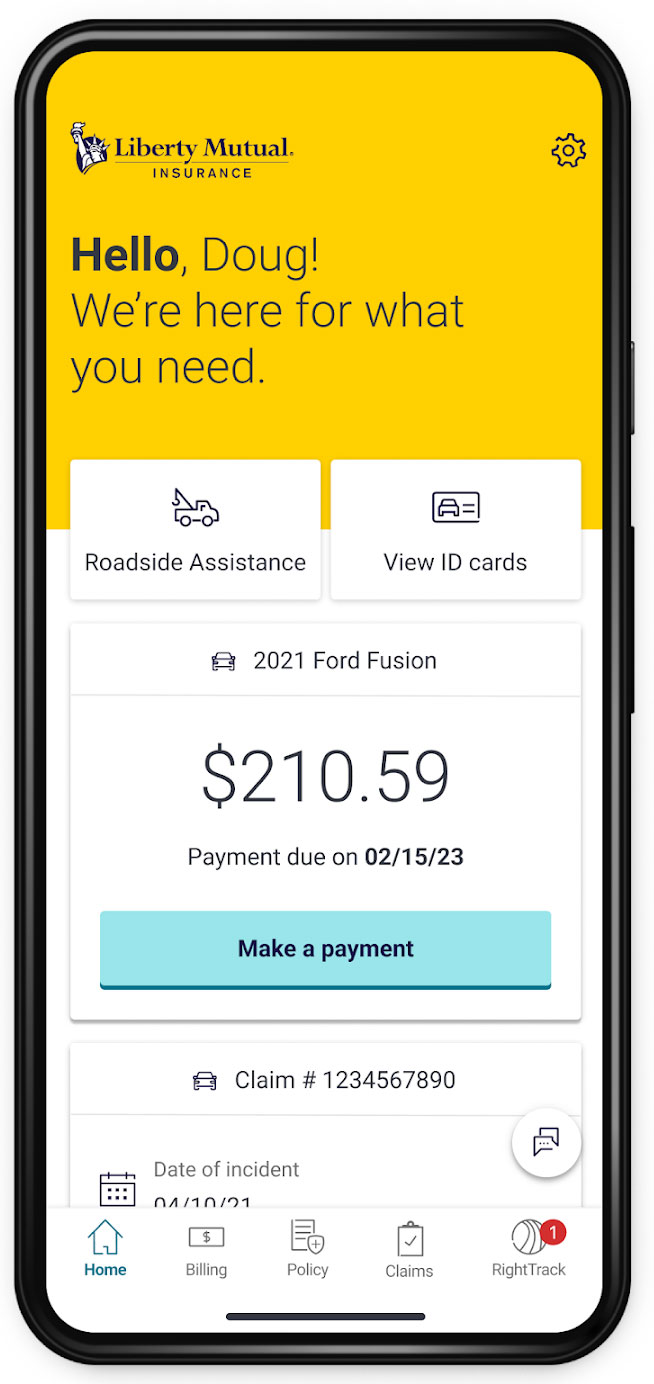The image displays a computer-generated graphic of a smartphone with the Liberty Mutual Insurance app open. The phone's design is unusually smooth and almost unrealistically black. The app interface features a bright mustard yellow header, with the Liberty Mutual Insurance logo, including the iconic Statue of Liberty symbol, positioned at the top left. Next to the logo, in bold black text, the app greets the user with "Hello, Doug, we're here for what you need," emphasizing the word "hello" in a bold typeface. A settings gear icon is located on the top right corner of the header.

Below the yellow header, two rectangular buttons are prominently displayed against a white background. The first button, labeled "Roadside Assistance," is accompanied by an icon of a tow truck, while the second button, labeled "View ID Cards," features an icon of an ID card. Dropping down further, there's a white rectangular section detailing a 2021 Ford Fusion, marked by a small car icon. This section indicates an outstanding payment of $210.59, which is due on 02/15/23, presented in bold black text.

A baby blue bar beneath this section offers a "Make a Payment" option in black text. Finally, at the bottom of the screen, another car icon is shown alongside a claim number, 1234567890, and a date of incidence, 04/10/21, which might be erroneously formatted. The overall graphic effectively highlights key functionalities of the Liberty Mutual Insurance app in a visually clear and organized manner.